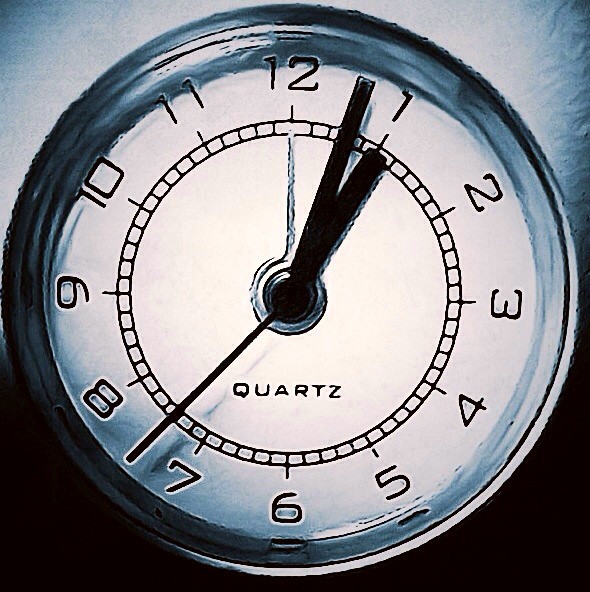The image depicts a zoomed-in, possibly distorted view of an artwork featuring the face of a round clock. The background transitions from white at the top to a very dark purple at the bottom. The clock has a silver edge and displays the numbers 1 through 12 in black around its circumference. Additionally, there is a circle of small squares running along the clock’s edge, marking each minute. The hour, minute, and second hands are also black and currently indicate the time as 3 minutes past 1 and 37 seconds. Beneath the clock hands, the brand "Quartz" is clearly visible. Though the image is in black and white, it seems to be a piece of decorative art, focalizing solely on the clock's face without any surrounding bands or additional text.